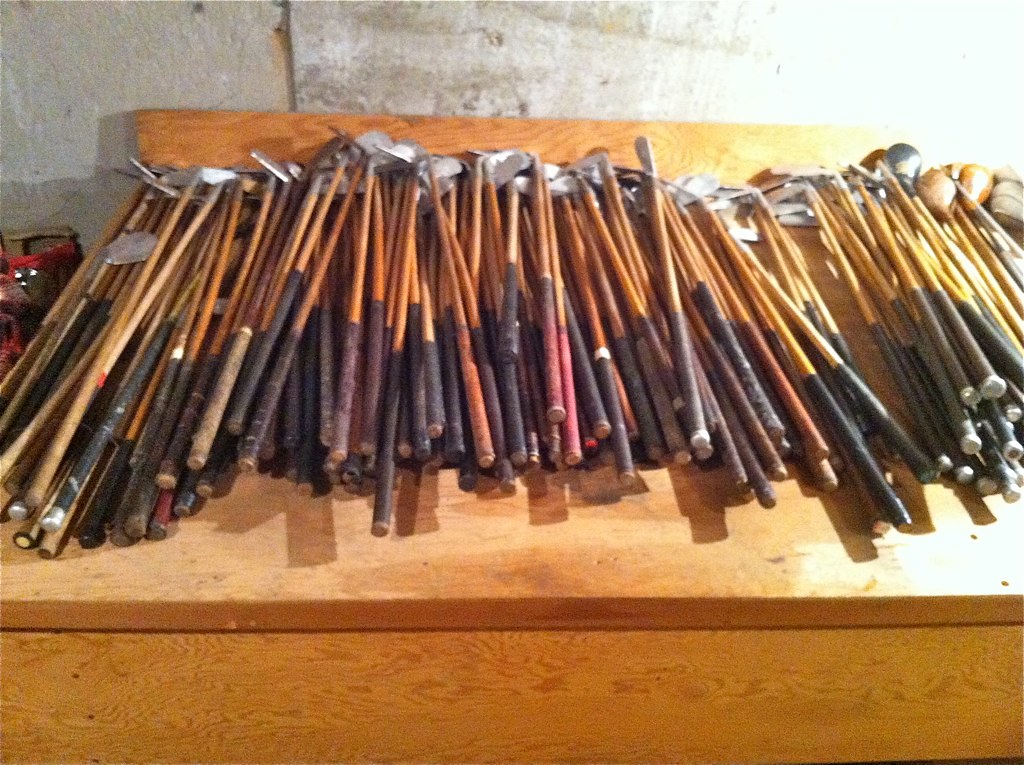In this detailed image, an assortment of tools, possibly garden implements or golf clubs, lie spread across a flat, light brown wooden bench. Each tool displays a shiny silver tip, while their handles vary in shade, with most presenting a yellowish to brown hue. The bottom halves of the handles, seemingly wrapped in black tape, darken further towards the grip. Among these handles, some display vibrant colors, including purple, red, and a single orange one, though most remain black. Towards the left and center of the image, a grayish stone or cement wall forms the backdrop, while it transitions to a light blue hue on the right. Additionally, to the far left, there is a small model of a red car, complete with headlights, perched on the bench. The image captures a sense of organized clutter, with dozens of these tools neatly arranged in rows, their heads consistently pointing towards the back.